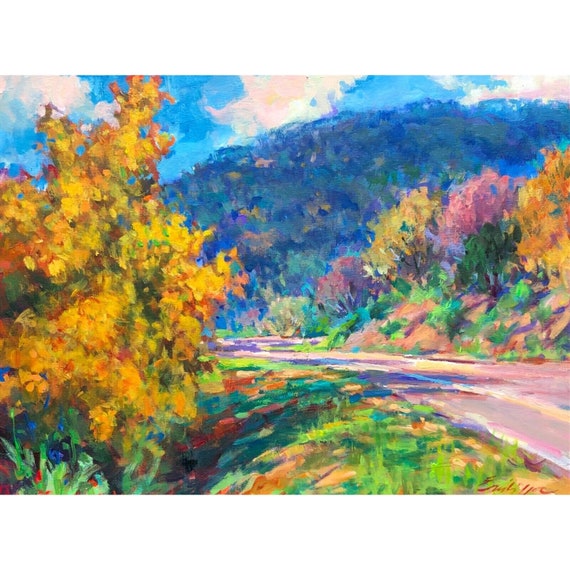Here is a detailed and cohesive caption combining elements from all three descriptions, with an emphasis on shared and repeated details:

"This vibrant painting, reminiscent of Van Gogh's style, depicts a winding country lane leading towards the foothills of a mountain range. The scene is set in autumn, characterized by the golden, peach, and pink hues of the trees lining the edge of the road. The grasses alongside display patches of brown, enhancing the seasonal feel. The sky above is fairly cloudy but retains more blue than white. The mountains in the background are rendered in various shades of blue, interspersed with pinks and golds, adding to the abstract quality of the painting. The road, which appears more modern due to a blurred yellow line, winds gracefully through the colorful landscape. The vibrant colors and enticing brushstrokes make this artwork a beautiful and captivating representation of a fall day."